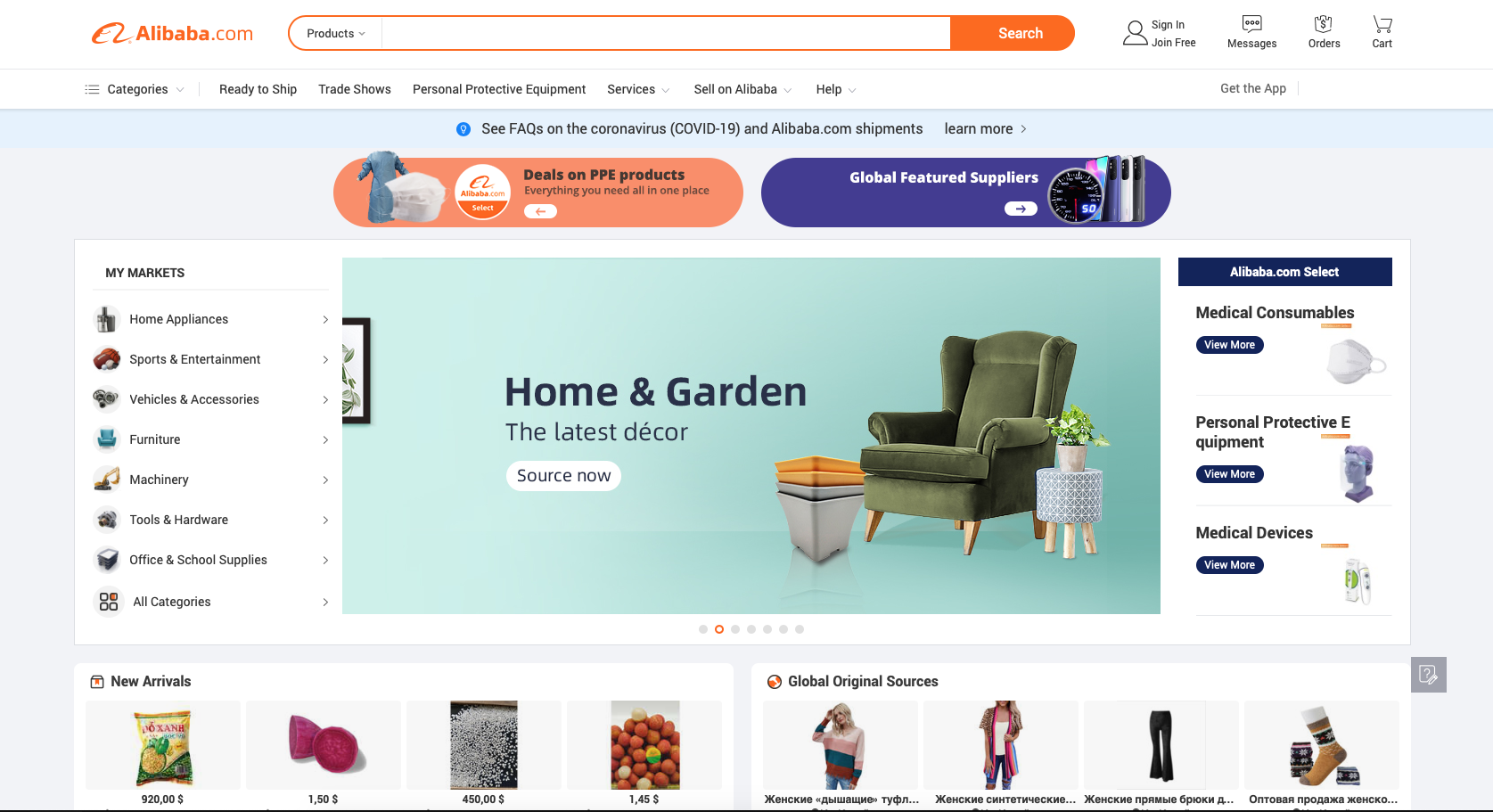This is a detailed description of a screenshot taken from the website Alibaba.com:

At the top of the screenshot, there is a white banner. On the top left corner, the company's name, "alibaba.com," is displayed. The "alibaba" part is in bold orange font, while the ".com" is in a regular font. Adjacent to the logo is a search bar, outlined with an orange oval. The search bar has a drop-down menu labeled "Products," followed by a wide open space for typing search queries. Attached to the right end of the search bar is a solid orange search button.

To the right of the main search area, there are several icons: "Join," "Messages," two other icons, and a cart icon, each with a small label underneath. All these elements are in small text.

Beneath the main white banner is a thinner white banner, separated by a small gray line. This banner features tabs labeled "Categories," "Ready to Ship," and five other options, though none of them appear to be selected. The text in this section is very small and blurry.

Below these banners is the main body of the webpage. This section starts with a banner that has a blue top and gray surroundings. It is divided into two large sections with an orange and a blue background, but the text inside these sections is too small to be read clearly.

Centered below this is a prominent image with a green background. The right side of the image features a sofa chair, and the left side displays the text "Home and Garden" with "the latest decor." Additionally, a white section at the bottom of the image includes a "Source Now" button. The image also features decorative elements like plants and tables in containers.

To the left of the main image is a column labeled "My Markets" with categories to choose from, such as "Home Appliances," "Furniture," and "Machinery." To the right of the image is another column with a blue top section, listing categories like "Medical Consumables," "Personal Protective," and "Medical Devices," each accompanied by a small picture.

At the very bottom of the webpage, there is a section titled "New Arrivals," showcasing four product images with prices underneath. Adjacent to this is another section labeled "Global Original Choices," also displaying four product images.

This detailed description encapsulates the various elements and structure present in the given screenshot from Alibaba.com.